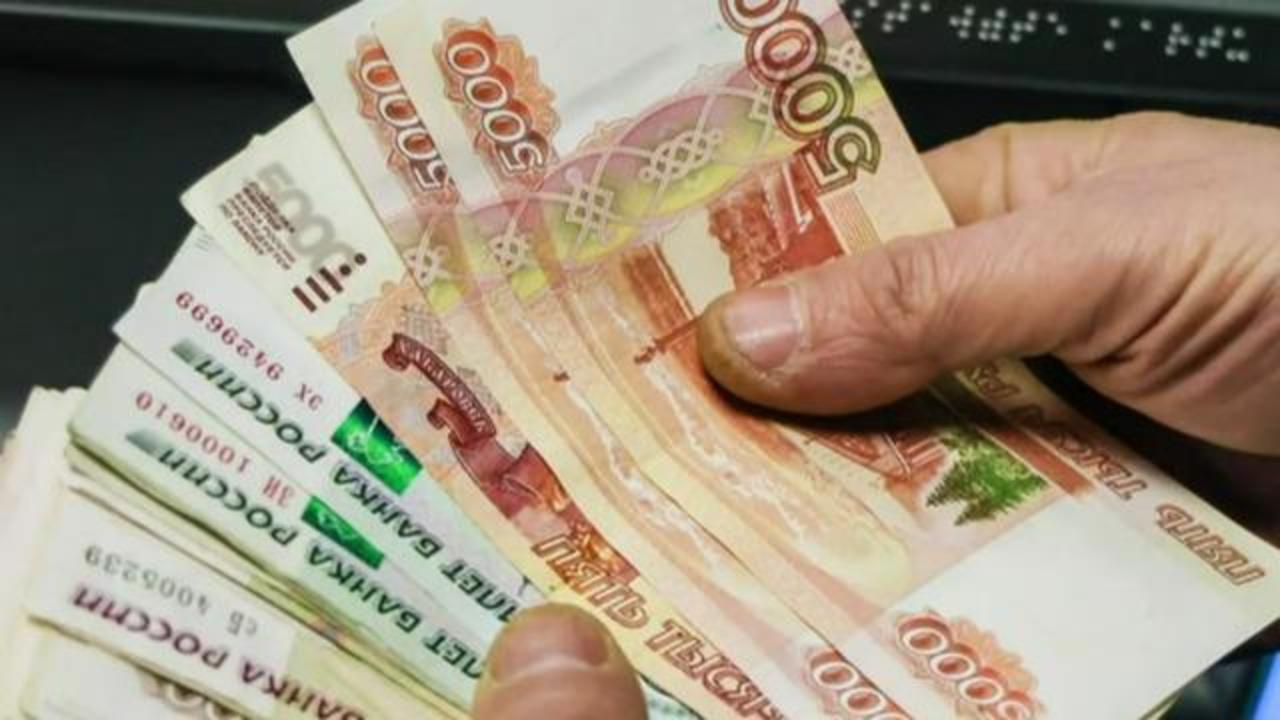The image is a close-up photograph of a pair of slightly wrinkled, older-looking hands holding a fanned-out stack of colorful foreign banknotes, likely Russian rubles, due to the Cyrillic script visible on them. The cropping is tight, showing only partial views of the hands and banknotes. The left thumb, just below the nail, is seen at the bottom left, while the right hand is more visible at the top right, with the thumb and part of the pointer finger extended. The three foremost banknotes prominently feature the number 5000 in white text against a red, bubble-like background, with additional green and yellow areas and white edges. Braille dots, white against a dark background, are noticeable in the top right corner, possibly on a black strip of photographed material.